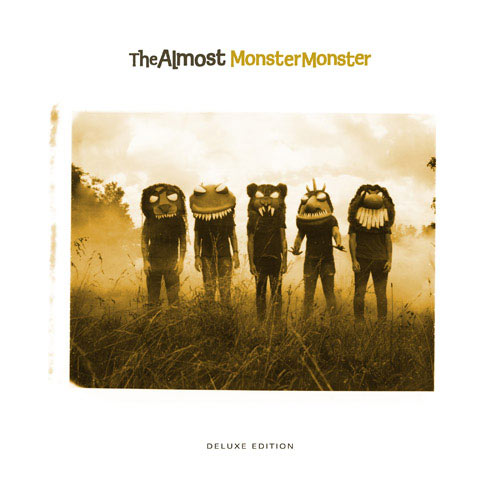The image appears to be an album cover featuring the words "The Almost" in black font and "Monster Monster" (all one word) in yellow font, with "Deluxe Edition" written in small black text at the bottom. Below the text, a photograph depicts five individuals, likely men, standing in a field. They are all wearing short-sleeved shirts, pants, and elaborate monster-like or animal masks with large protruding teeth and eerie white eyes. The color scheme of the image is primarily a golden yellowish-green, with an overall effect that resembles a black-and-white photo enhanced with tans and hints of color. The setting seems rural, possibly reminiscent of a Midwestern town with lots of open space, and distant trees are visible behind a hazy mist or dust that obscures parts of the figures' legs. The weather appears bright and cloudy, contributing to the almost surreal, artful atmosphere of the scene, suggestive of an art project or artistic concept.